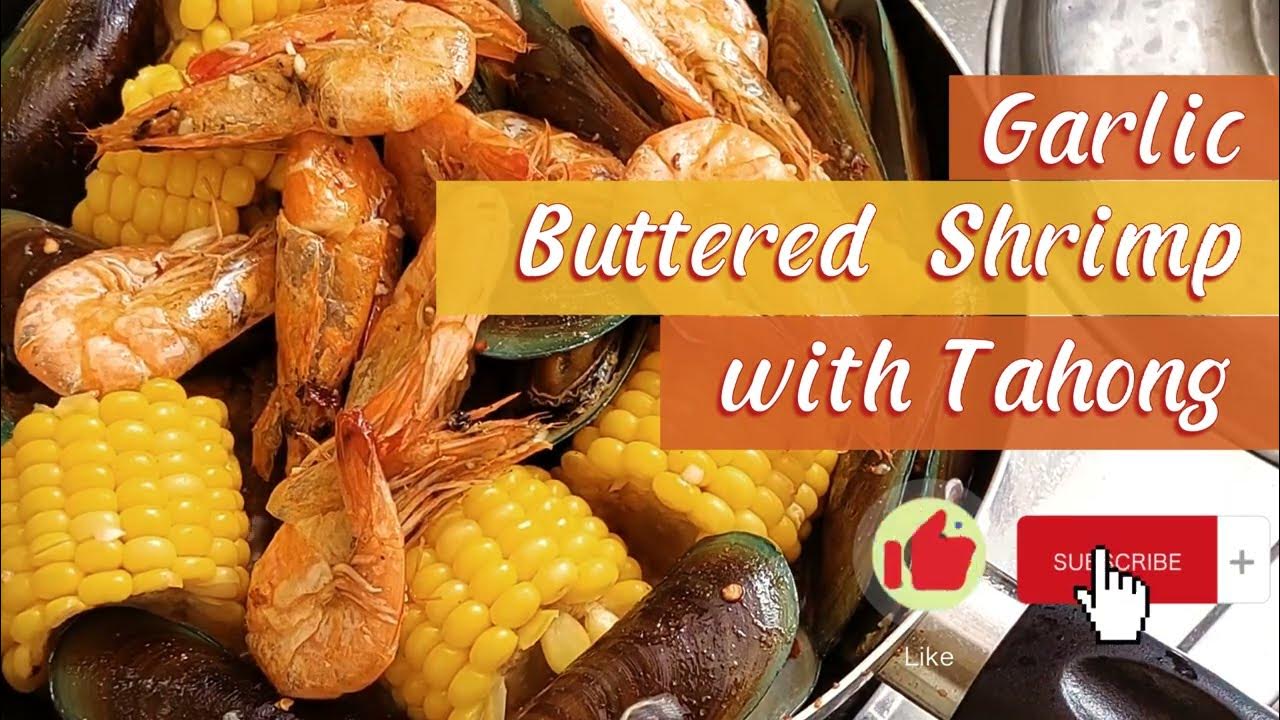This image appears to be a screenshot from a YouTube video showcasing a recipe for "Garlic Buttered Shrimp with Tahong." The recipe title is prominently featured on the right side of the image, with "Garlic" on an orange background, "Buttered Shrimp" on a yellow background, and "with Tahong" again on an orange background, all in white font. Below the title is the word "subscribe" in white on a red background, with a plus sign next to it. A pointer finger icon is poised over the subscribe button. To the left of the subscribe button is a red thumbs-up icon on a green background with the word "like" written beneath it, indicating user engagement features commonly seen on YouTube.

On the left side of the image, the photo of the meal displays a vibrant assortment of cooked ingredients, suggesting a seafood boil or a similar dish. There are about seven or eight whole shrimp displaying a coral pink hue, alongside cooked pieces of corn on the cob, approximately one and a half inches long, showcasing a rich yellow color. Additionally, there are mussels with brown shells and a greenish edge, indicating they might be tahong, as the dish name suggests. All of these ingredients are presented in a steel pot or pan, emphasizing the rustic and hearty nature of the seafood dish.